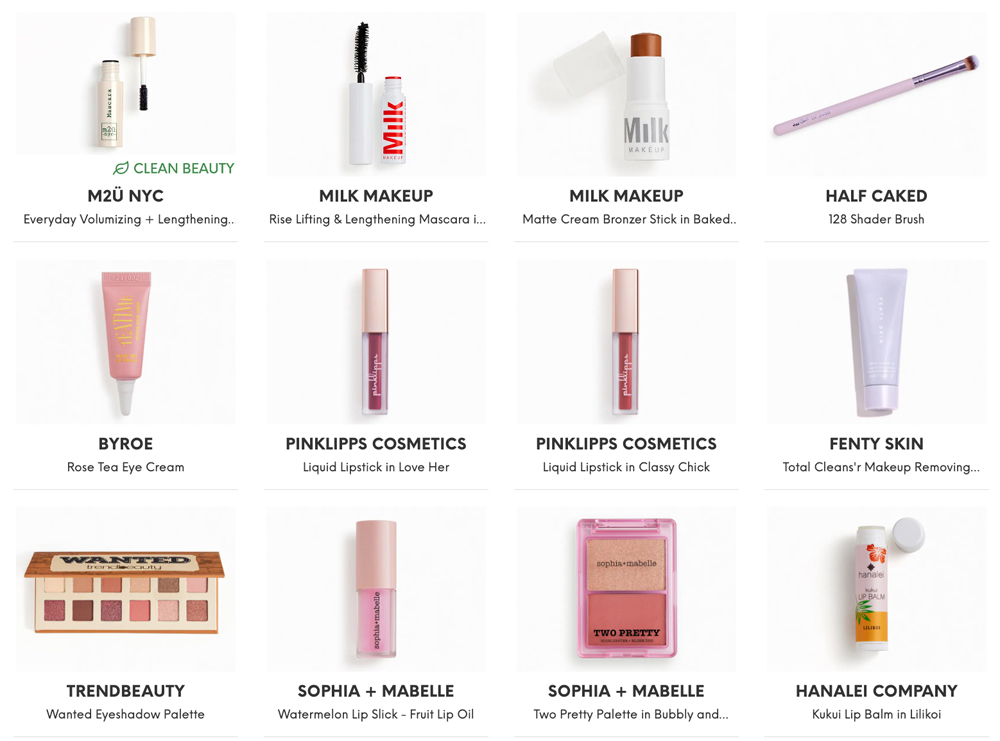This image showcases a diverse collection of makeup products arranged in a neat grid formation with three rows and four items in each row.

- **Top Row, First Item:** "Clean Beauty - M2U NYC Everyday Volumizing + Lengthening Mascara." The product packaging is showcased with the name labeled below, along with a brief description emphasizing its volumizing and lengthening properties.
- **Top Row, Second Item:** "Milk Makeup - Rise Lifting and Lengthening Mascara." The mascara is prominently displayed with its name and a succinct description beneath it, which highlights its lifting and lengthening capabilities.
- **Top Row, Third Item:** "Milk Makeup - Matte Cream Bronzer Stick in Baked." This item features the bronzer stick with its name and a short description detailing its matte finish and creamy texture.
- **Top Row, Fourth Item:** "Half Caked - 128 Shader Brush." The brush is presented with its name and a brief description, likely focusing on its uses for eyeshadow application.

- **Middle Row, First Item:** "BYRO - Rose Tea Eye Cream." The eye cream is visually represented with its name and a description, possibly detailing its soothing and hydrating effects.
- **Middle Row, Second Item:** "Pink Lips Cosmetic - Liquid Lipstick in Love Her." This liquid lipstick is displayed with its name and a brief description that might emphasize its color and longevity.
- **Middle Row, Third Item:** While left incomplete, it can be inferred this is another product from Pink Lips Cosmetic, likely another variant of their liquid lipstick.

For a vivid understanding, each item features clear images, detailed names, and concise descriptions, ensuring the viewer can easily identify and understand each product's purpose and characteristics.